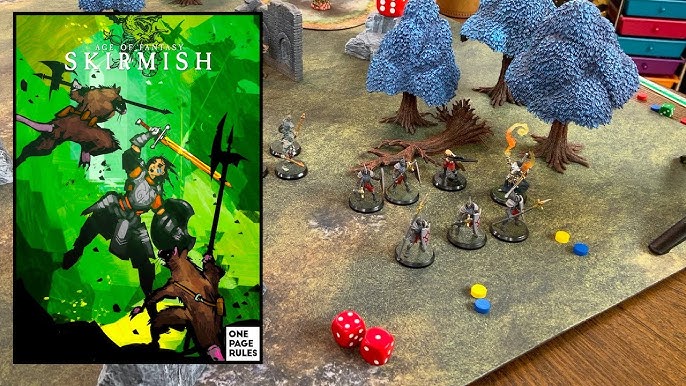The photograph captures a Dungeons & Dragons-style dice game set on a richly detailed board designed to resemble a forest, lying atop a brown wood table. The playing board features a lifelike forest scene, populated with miniature figurines of knights positioned in front of trees with brown trunks and distinct blue leaves, located in the upper-right corner. Notably, red dice with white dots displaying the numbers 5, 4, and 1 are scattered across the bottom portion of the board. Additionally, the scene includes small yellow and blue cylindrical objects, resembling buttons or discs, placed near the figures.

In contrast to the realistic board, the left-hand side of the image displays part of an overlaid comic-style cover from a rulebook, "Age of Fantasy Skirmish," against a green background. This cover features an illustration of a knight battling two mutant rat creatures. Text in the lower right corner of the cover reads "One Page Rules," indicating the game's name and ruleset. The overall scene beautifully blends detailed lifelike elements with stylized graphic art, creating a vivid and engaging snapshot of the game setup.